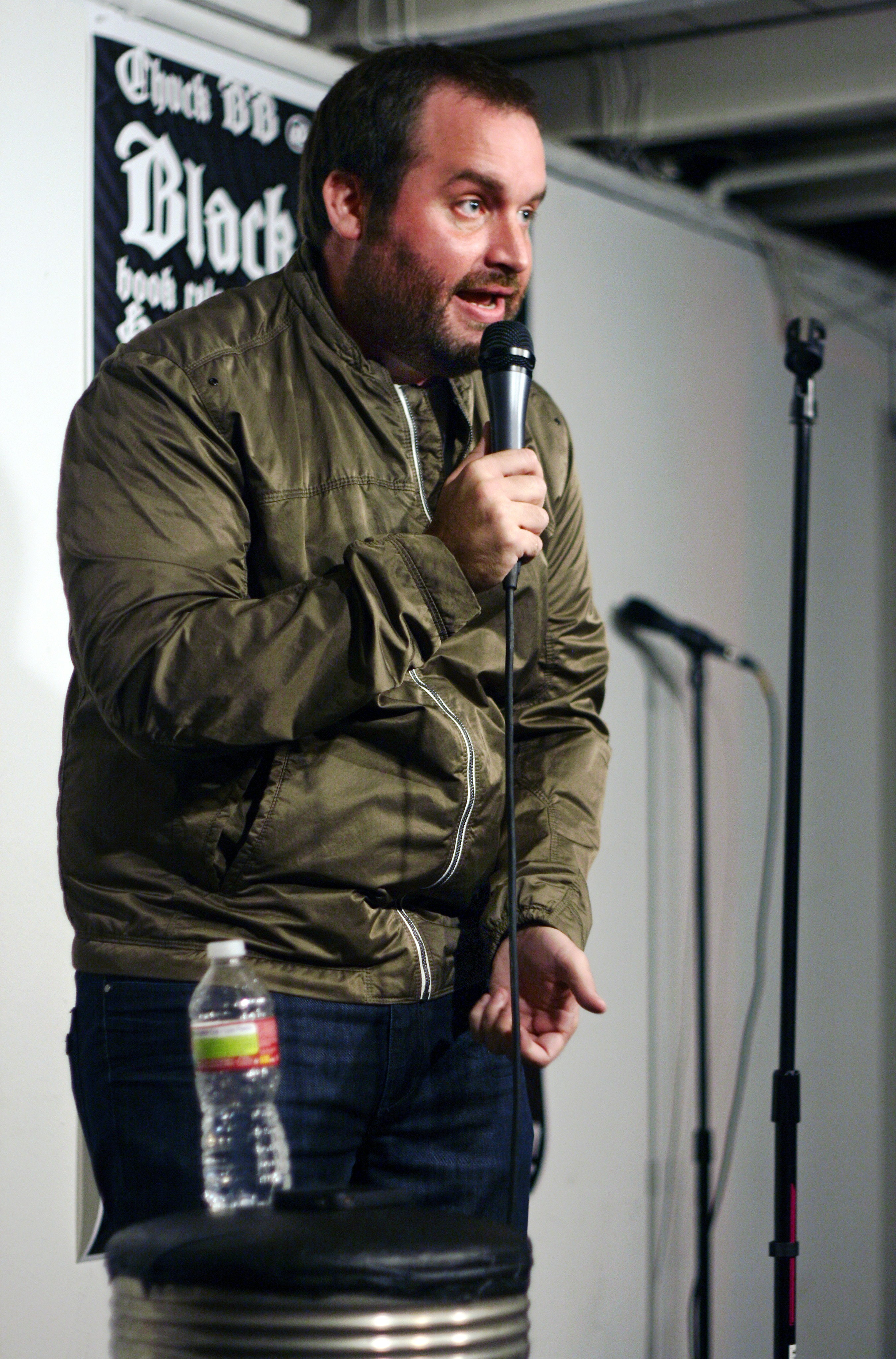In this color photograph, a man stands on stage, appearing to address an audience with a wired microphone in hand. He is gazing towards the crowd, seemingly in the midst of speaking, which suggests he could be a comedian performing his act rather than giving a formal speech. The man is dressed in dark blue denim jeans and a light green or olive windbreaker jacket that reaches his waist. He has a medium Caucasian appearance, possibly Mediterranean, with a small beard, a slightly receding hairline, dark brown hair, and brown facial hair. He is slightly overweight. To his right, a black microphone stand with adjustable knobs is visible, and another wired microphone rests against the wall behind him. Directly in front of him is a black leather-topped round stool, holding a small plastic water bottle with a red tag. The backdrop is a black wall with a black poster attached to it, reinforcing the intimate and possibly comedic atmosphere of the setting.